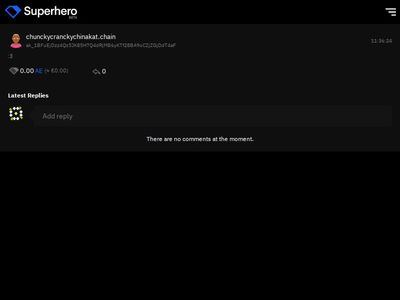Screenshot of a website displaying a "Superhero" header. In the top right corner, three horizontal bars act as a menu icon. On the page, a profile picture of a girl wearing a pink shirt is visible. To the immediate right of the profile picture is small text, possibly reading "11 of 14." The page features a section titled "Latest Replies." The background is predominantly black, with a gray rectangle containing the text "Add reply" in light gray font. Additionally, there's a black rectangle with white lettering stating, "There are no comments at the moment."